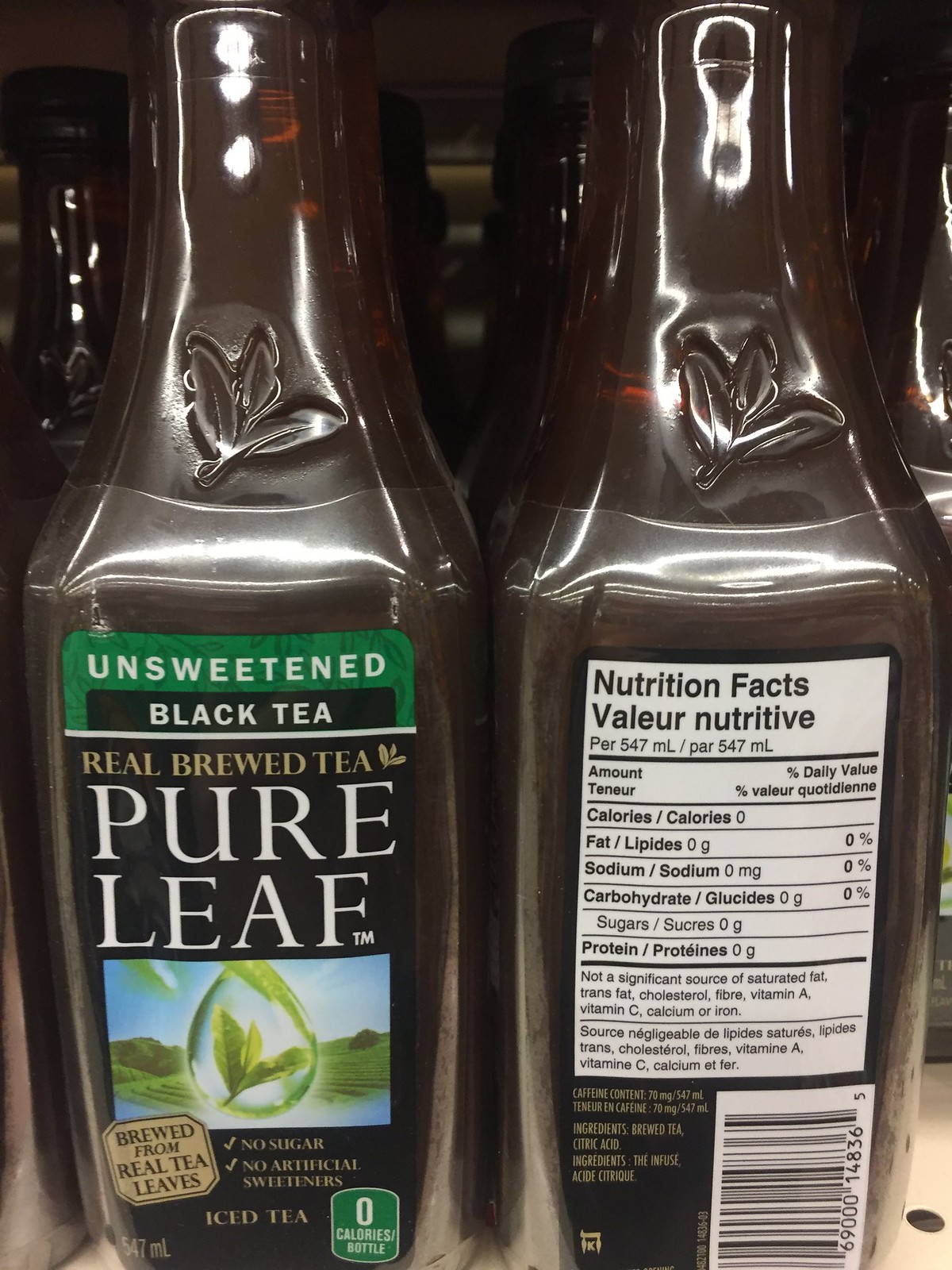In the image, two bottles of Pure Leaf Black Tea are positioned side by side. The bottle on the left prominently displays the front label, which identifies the tea as unsweetened black tea under the Pure Leaf brand. A crisp, green tea leaf serves as part of the label's design, symbolizing the product's natural ingredients. The bottle on the right showcases the nutritional facts. These details are provided in both English and another language, highlighting essential nutritional information: zero calories, zero sugar. Below the nutritional facts section, the list of ingredients is clearly printed, followed by a barcode at the bottom. The well-organized presentation offers a comprehensive view of both the branding and nutritional content.